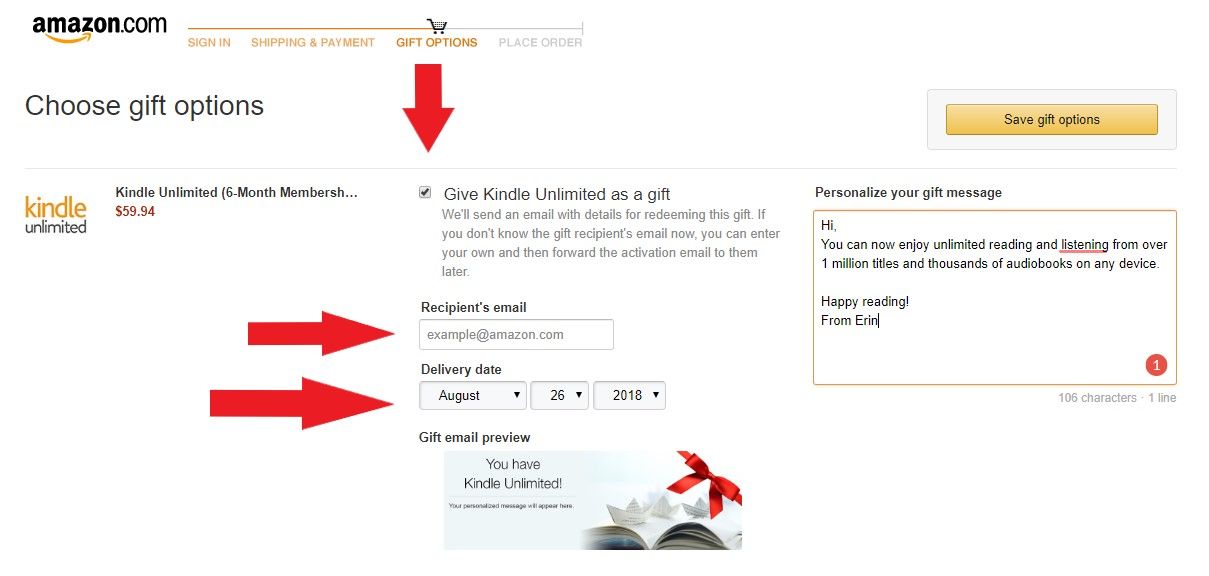The image is a screenshot from the website amazon.com, featuring a predominantly white background. In the upper left corner, the iconic Amazon logo is displayed with its characteristic orange swoosh. Adjacent to the logo, there is a horizontal navigation bar divided into sections marked by gray and yellow colors, indicating steps in the purchasing process: "Sign In," "Shipping and Payment," "Gift Options," and "Place Order." 

Directly above the "Gift Options" section, there is a small shopping cart icon. An adjacent red arrow points downward with the text "Choose Gift Options" beside it. To the right of this section, a yellow button is labeled "Save Gift Options."

Below the main navigation, yellow text reads "Kindle Unlimited," followed by "Kindle Unlimited Six Month Membership" in regular font. The price, "$59.94," is prominently displayed in red. To the right, two red arrows highlight the phrase "Give Kindle Unlimited as a Gift."

Further down, the form fields labeled "Recipient's Email," "Delivery Date," and "Gift Email Preview" are visible. On the right side of these fields, a yellow box instructs the user to "Personalize your gift message."